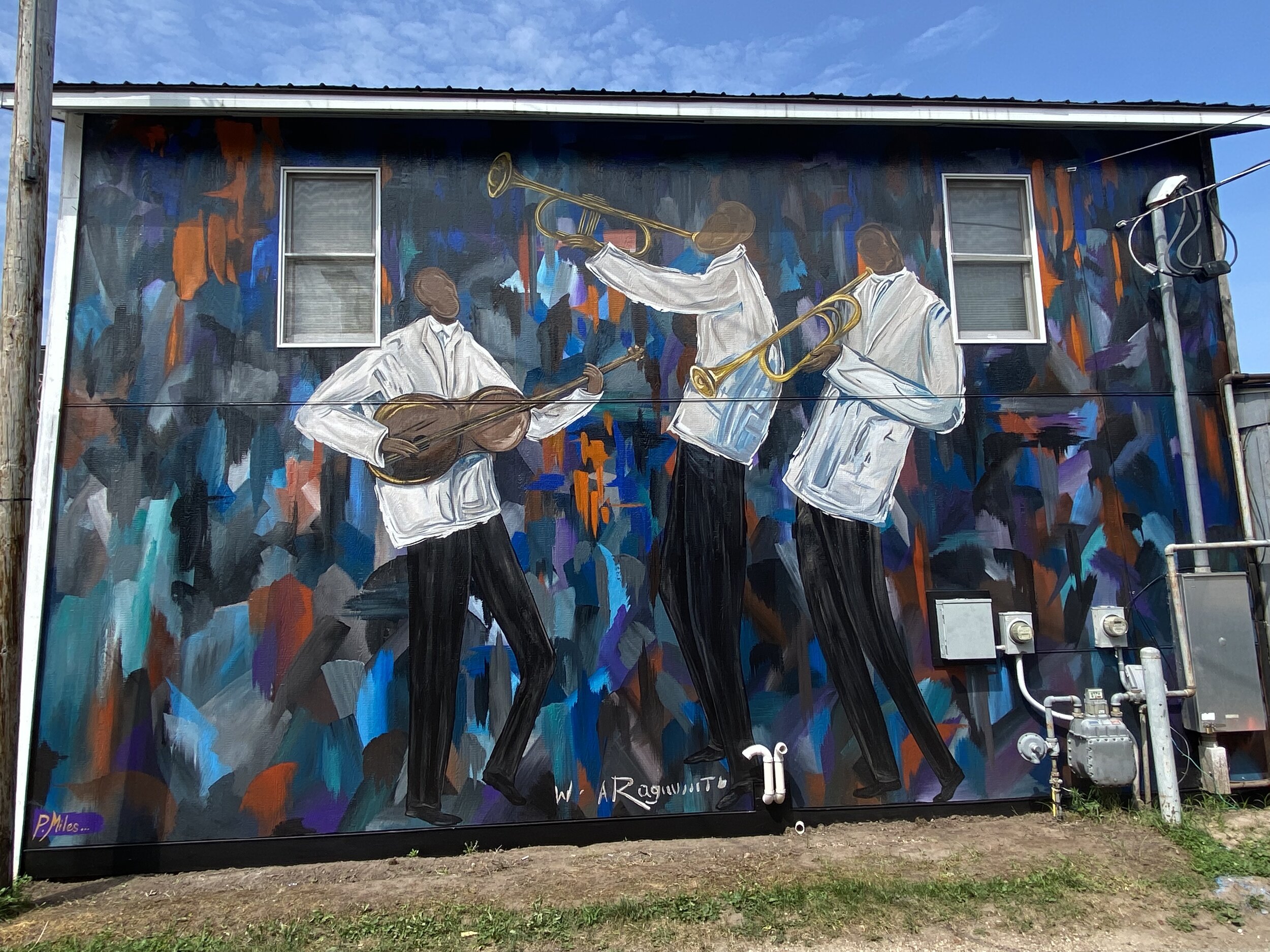The image captures a vibrant mural painted on the side of a building. The mural spans the entire wall, featuring an abstract background in dark, jewel-toned colors including dark orange, blue, black, teal, cobalt blue, red, gray, purple, and light blue. The focal point of the mural is a jazz trio composed of three dark-skinned men, all wearing white shirts, white jackets, black pants, and black shoes. Two of the men are playing trumpets, while the third is playing a guitar-like instrument. The building itself has two white windows with two glass panels each, and various electrical meters and wires are attached to its side. The grass below the mural is mostly dead, with a strip of green. The mural is signed by the artist, W. Araguntia, although the signatures are not entirely legible.